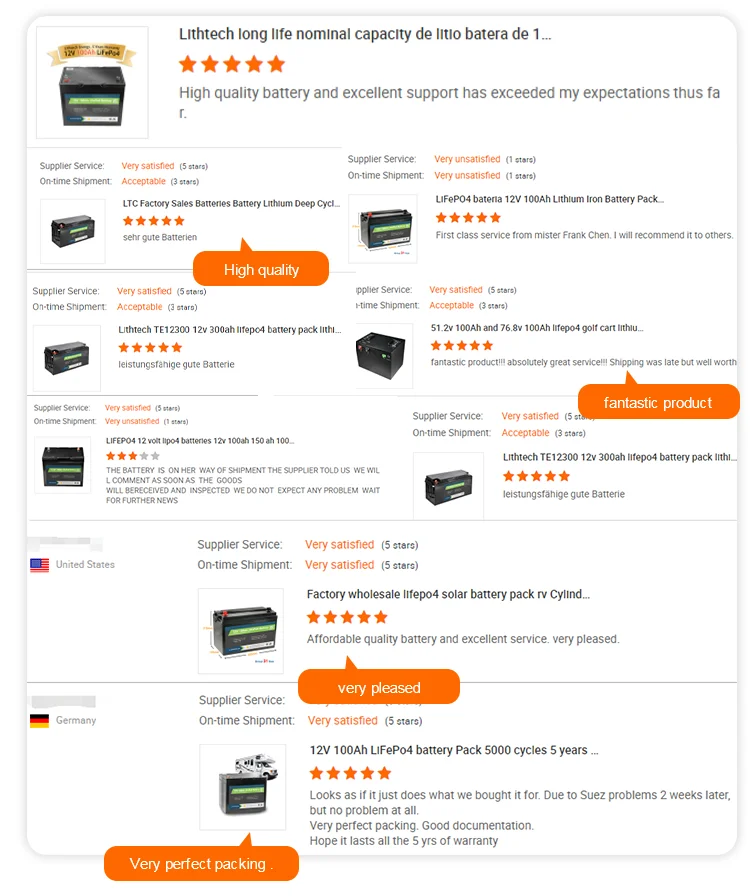The image displays an array of product reviews and descriptions, primarily focused on a high-quality lithium battery pack. At the top of the image, there is a blurry piece of text with the word "Lithtech" prominently visible. Other phrases such as "long life" and "nominal capacity" are also noticeable but somewhat obscured.

The main subject of the reviews is the "D-something" model battery, which has garnered high praise and five-star ratings across various feedback snippets. The description "high-quality battery and excellent support has exceeded my expectation thus far" is partially visible, followed by an incomplete phrase.

Several orange text boxes provide additional positive feedback. One of these boxes reads "high-quality lithium battery pack," and another one mentions "fantastic product." A separate orange box highlights that the product is sold at "factory wholesale," with an emphasis on it being a "solar battery pack" rated five stars.

Additional reviews applaud the product's portability and quality, stating "excellent service, very pleased." Another orange box underscores buyers' satisfaction with the phrase "very perfect packing."

Overall, the image is a montage of glowing reviews and attributes for a top-tier lithium battery pack, marked by high ratings and commendations for both the product's quality and the service provided.